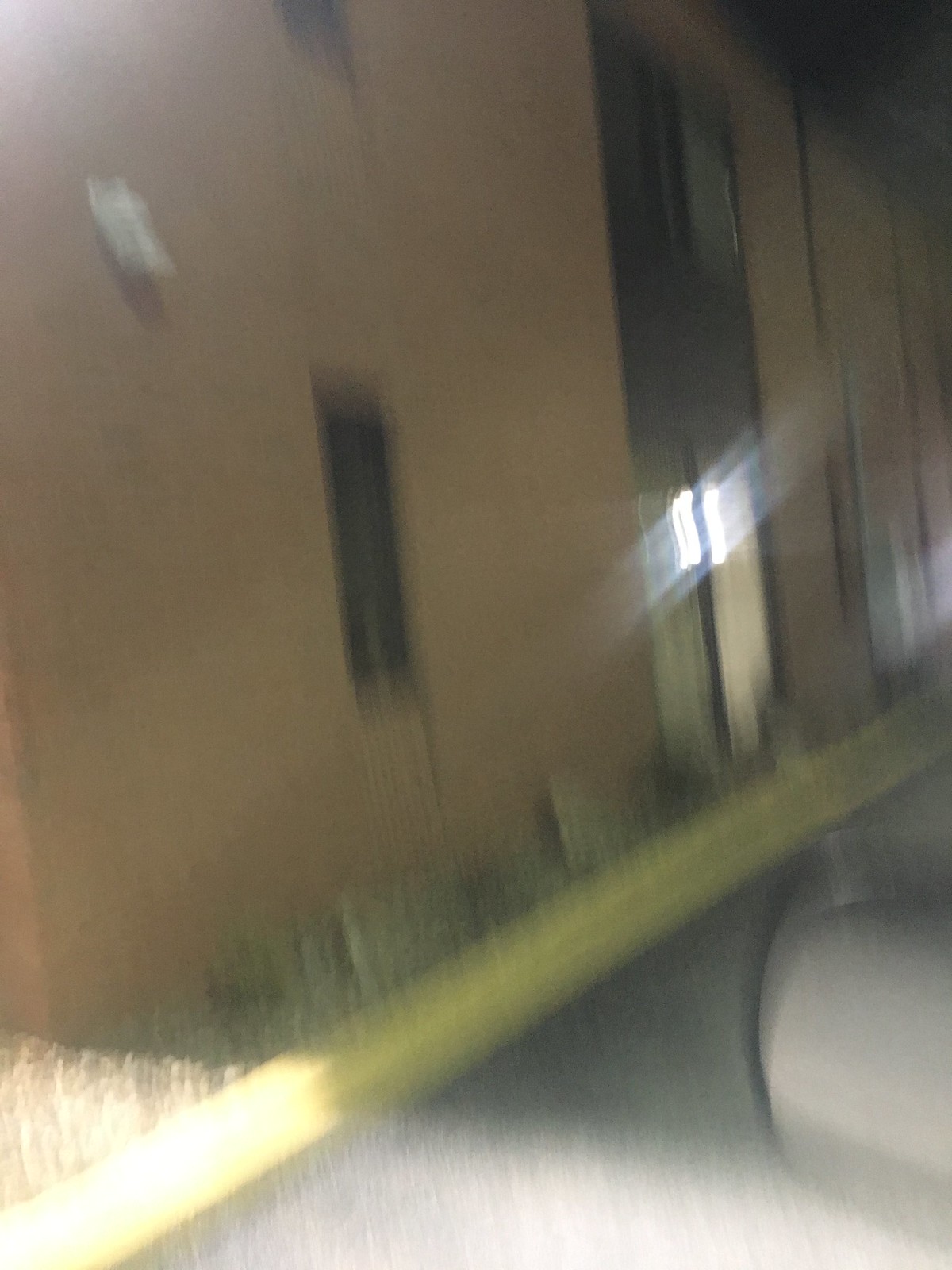This blurry nighttime photo, taken from inside a moving car, features a brown brick building that resembles a dormitory. The car's rearview mirror is faintly visible in the lower right corner. The image captures a grey paved road with a yellow curb running diagonally from the lower left to the center right edge. In front of the building, there is a mix of green foliage and brown gravel. The building itself has a series of windows; two sets on the upper floor and two on the lower floor, some of which may form a larger divided window or door. A light source outside the frame illuminates the scene, with additional light filtering through the first-floor windows, creating rectangular reflections. A white object, possibly a vent, is attached to the building, and a plastic bag is caught mid-air next to it. The overall photo is blurred, with minimal details sharply defined.